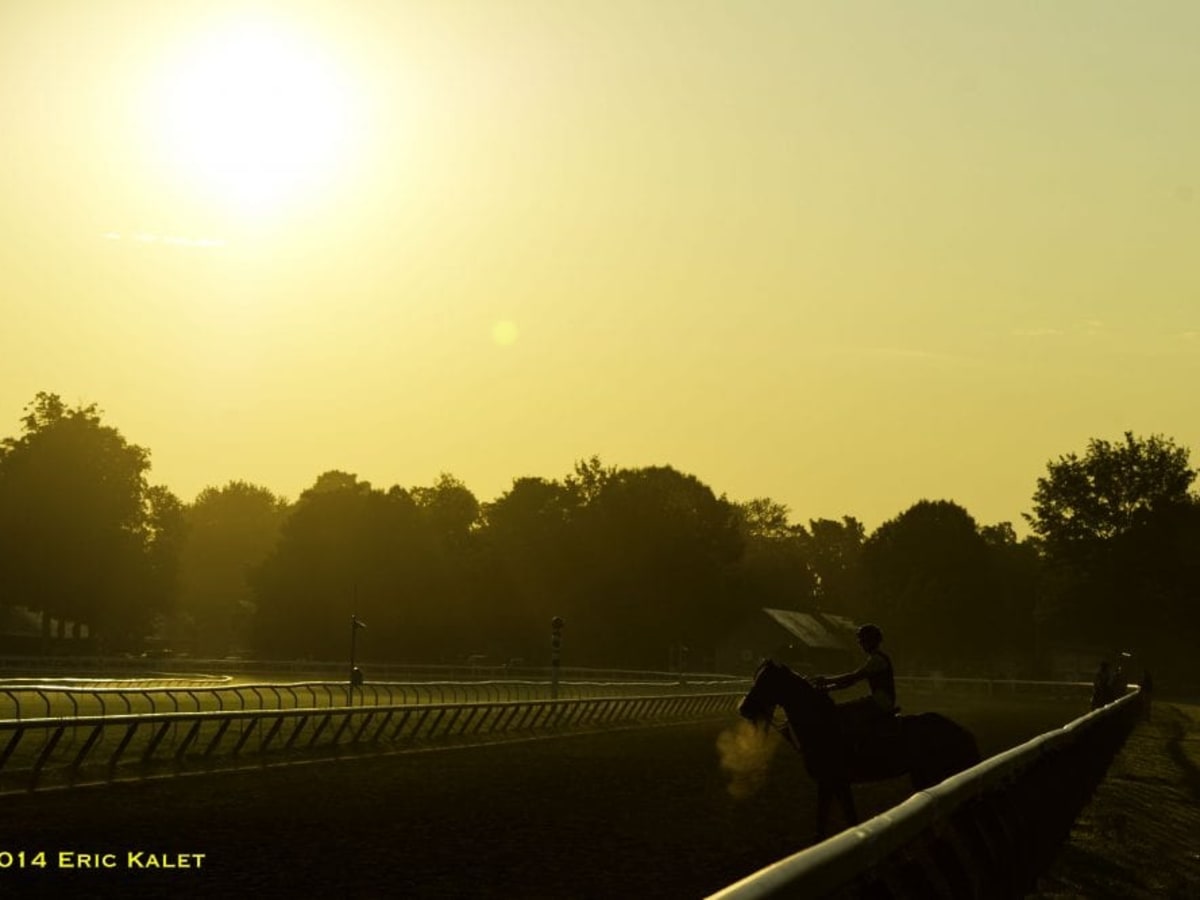The image depicts a scene at a horse racing track during what appears to be early morning or late afternoon based on the beautifully colored sky. The sky is a gradient of vibrant hues transitioning from bright white around the sun, situated in the top left corner, to deep oranges, yellows, and even hints of green and teal toward the top right. Dominating the background is a dark tree line rendered as mere shadows, adding depth to the picture.

In the lower portion of the image, a racetrack is visible, marked by both inner and outer railings. The track appears dark, almost black, against the brightly lit sky. A single horse, carrying a jockey, stands on the track near the bottom right, facing the inner railings. Both the horse and the jockey appear as black silhouettes, adding to the dramatic contrast. A notable detail in the image is the possible breath vapor visible under the horse's nose, indicating a cold atmosphere.

In the lower left corner of the image, the text "014 Eric Calais" is prominently displayed in yellow letters, potentially identifying either a location or an event related to the scene captured. No other people, animals, vehicles, or additional text are present in the image, keeping the focus on the lone horse and its rider against the vivid, colorful sky.